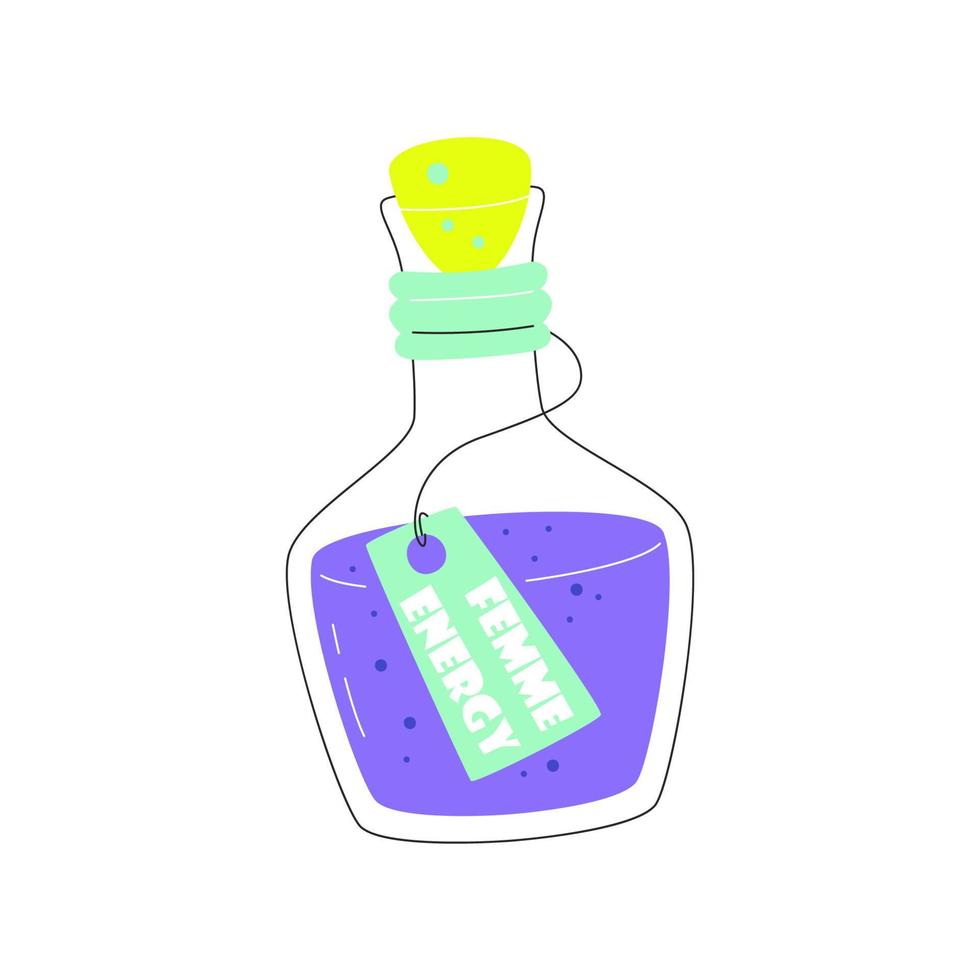The image depicts a detailed digital drawing of a small glass bottle, showcasing a simplicity yet vibrant cartoony style. The clear bottle, resembling more of a perfume bottle with its wider base and thinner neck, contains a blue liquid that fills about three-quarters of the bottle. Floating in the liquid are blue bubbles, adding a dynamic element to the illustration. The bottle’s neck is adorned with a green string tied just below a yellow cork, from which hangs a light green rectangular tag. The tag prominently displays the words "Femme Energy" in bright white letters, making it a focal point of the image. Against a plain, pure white background, the bottle stands out with its colorful and concise elements, creating a striking contrast that highlights the playful and charming nature of the design.